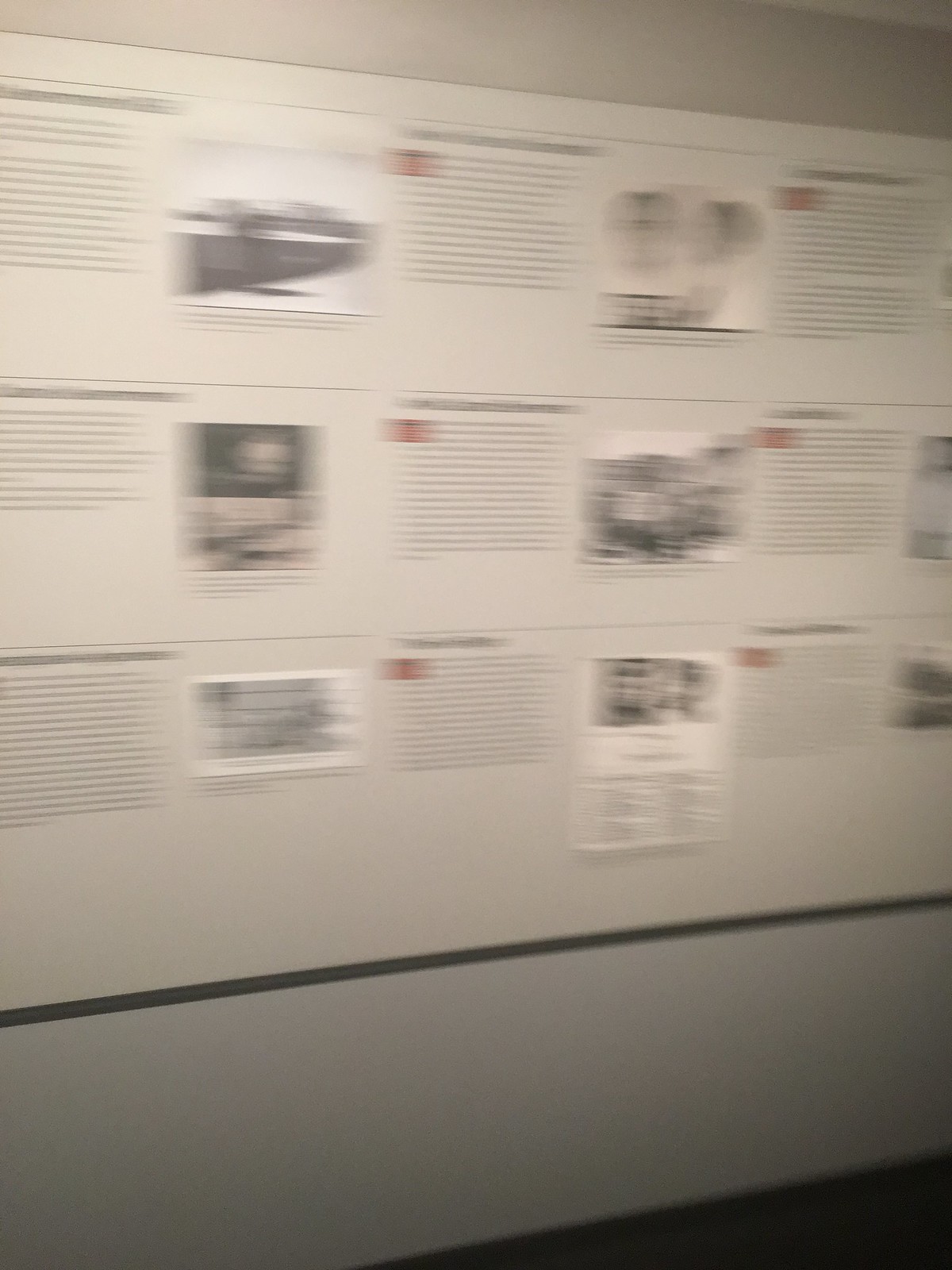This blurry vertical photograph depicts a white-gray wall taken at a slight angle from bottom left to upper right, likely in an interior museum setting. Dominating the wall is a large white display board made up of nine sections, organized into three rows and columns. Each section on the display appears to feature an arrangement of text and images, with three to four pieces of information visible in each row, although the blur makes the content indistinguishable. Notably, some sections contain black-and-white photographs accompanied by paragraphs of black text, while others have red rectangles in the upper left corners. Below the display, a black line spans horizontally across the wall. The lower part of the wall transitions to a lighter gray and the dark-colored floor is faintly visible. The overall image quality is compromised due to low light and a slow shutter speed, rendering the detailed information unreadable.